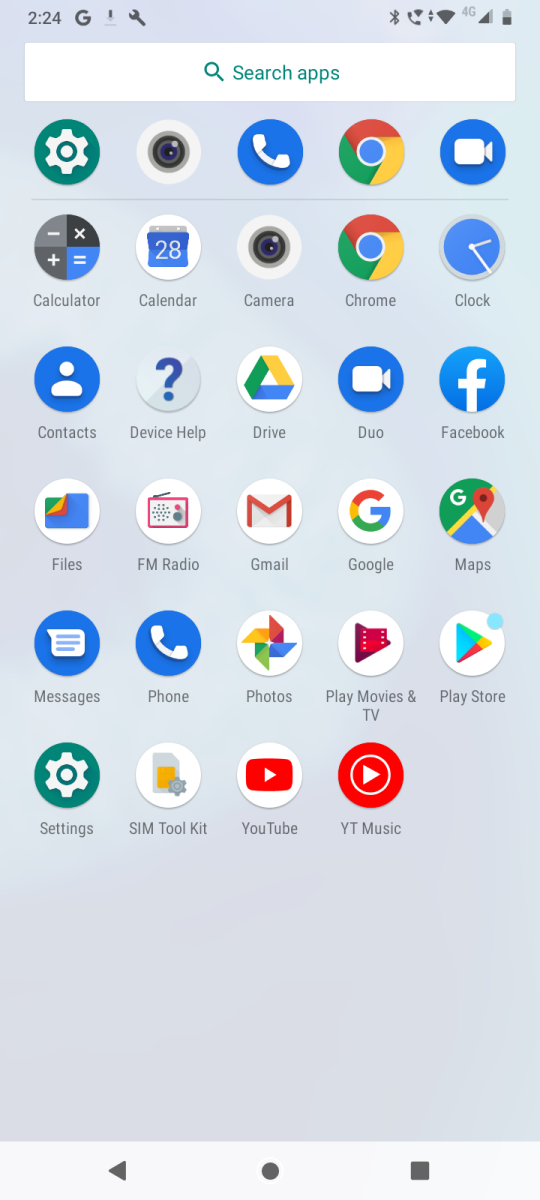A detailed image of an Android smartphone’s main screen is shown. The phone displays a variety of app icons organized in a grid layout. At the top of the screen, there is a "Search Apps" bar. Visible apps include YouTube, YouTube Music, SIM Toolkit, SM Toolkit, Settings, Play Store, Play Movies, Photos, Phone, Messages, Files, FM Radio, Gmail, Google Maps, Facebook, Duo, Drive, Device Help, Calculator, Contacts, Chrome, and Camera.

In the status bar at the very top, several icons indicate the device's current status: battery level, active Wi-Fi connection, Bluetooth enabled, and location services turned on. Additionally, the phone appears to be engaged in a call and is in the process of downloading something, as suggested by the presence of a call icon and a download indicator. There is also a small wrench icon and the Google logo, suggesting tools or updates and Google services.

The background of the screen is solid black, enhancing the visibility of the app icons and status indicators. At the bottom of the screen, the familiar Google Navigation buttons are displayed: Multitask, Back, and Home buttons, providing easy access to essential navigation functions.